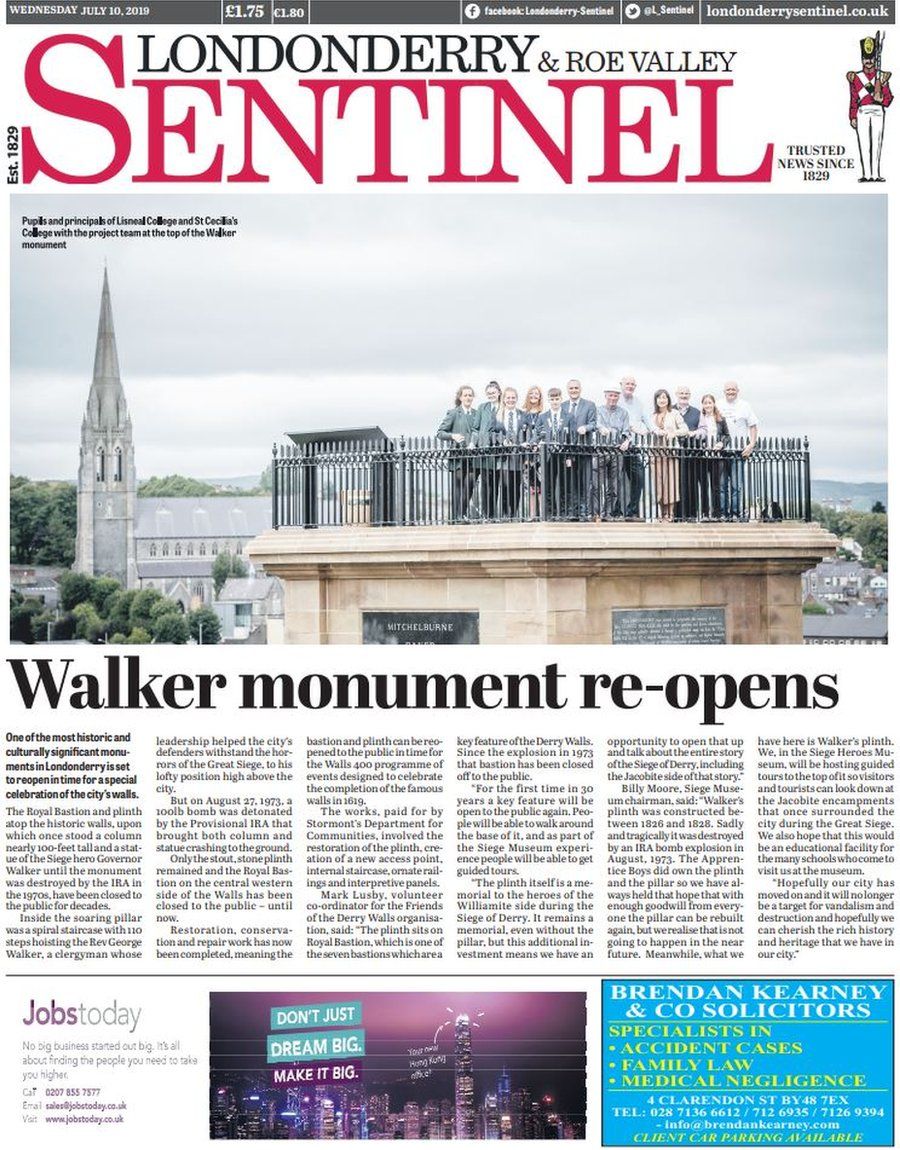This is a detailed caption for the provided image:

---

The front page of the newspaper features the headline "Londonbury and Rho Valley Sentinel," with "Sentinel" prominently displayed in very large red letters. To the far right of the header, there is an image of a soldier resembling a traditional British soldier. Just below the title, a large photograph showcases a group of people standing on top of a building, congregating in a small open area. Beneath the photo, the bold black caption reads, "Walker Monument Reopens," signaling a significant event. The article detailing this event is positioned below the caption. 

In the bottom left corner of the page, there is a section titled "Jobs Today" in purple font, offering employment opportunities. Centrally located at the bottom, there is a rectangular photograph of a sprawling cityscape with an inspiring text overlay that reads, "Don't just dream big, make it big." To the right of this image sits a small square advertisement, characterized by a blue background and white and yellow text. 

Additionally, diagonally at the top, positioned at the bottom of the letter "S," there is a small vertical black font inscription stating, "Established 1829."

---